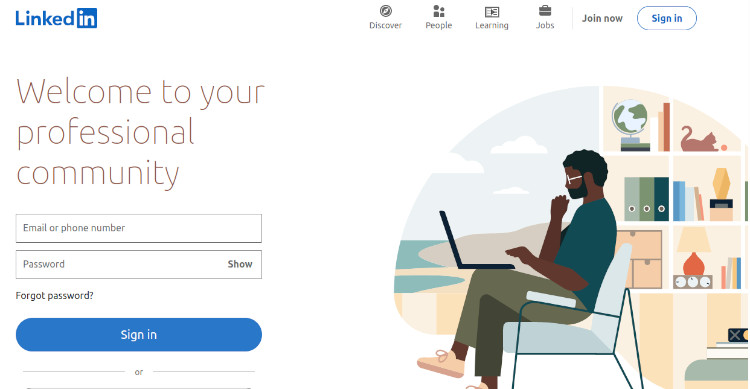This image captures the LinkedIn sign-in page. In the upper left corner, the LinkedIn logo is prominently displayed. The "LinkedIn" text is in blue, with the "IN" enclosed in a blue square with white font, linked together through the "L" forming an elegant continuation. To the right of the logo, there is a significant blank space, followed by a navigation menu. The menu includes buttons for "Discover," "People," "Learning," and "Jobs."

On the far right of this bar, there are options for user engagement: a "Join now" button followed by a "Sign in" button, outlined in blue with a white background and blue text.

Beneath the logo and navigation bar, there is a welcoming message, slightly left-justified, saying "Welcome to your professional community." This message is broken into three lines: "Welcome to your," "professional," and "community."

Below this greeting, there are input fields for user credentials. The first field is for the email or phone number, followed by a second field for the password. A "Forgot password?" link is in small font just below the password field. At the bottom of this section, there is another "Sign in" button, encouraging users to log in to their accounts.